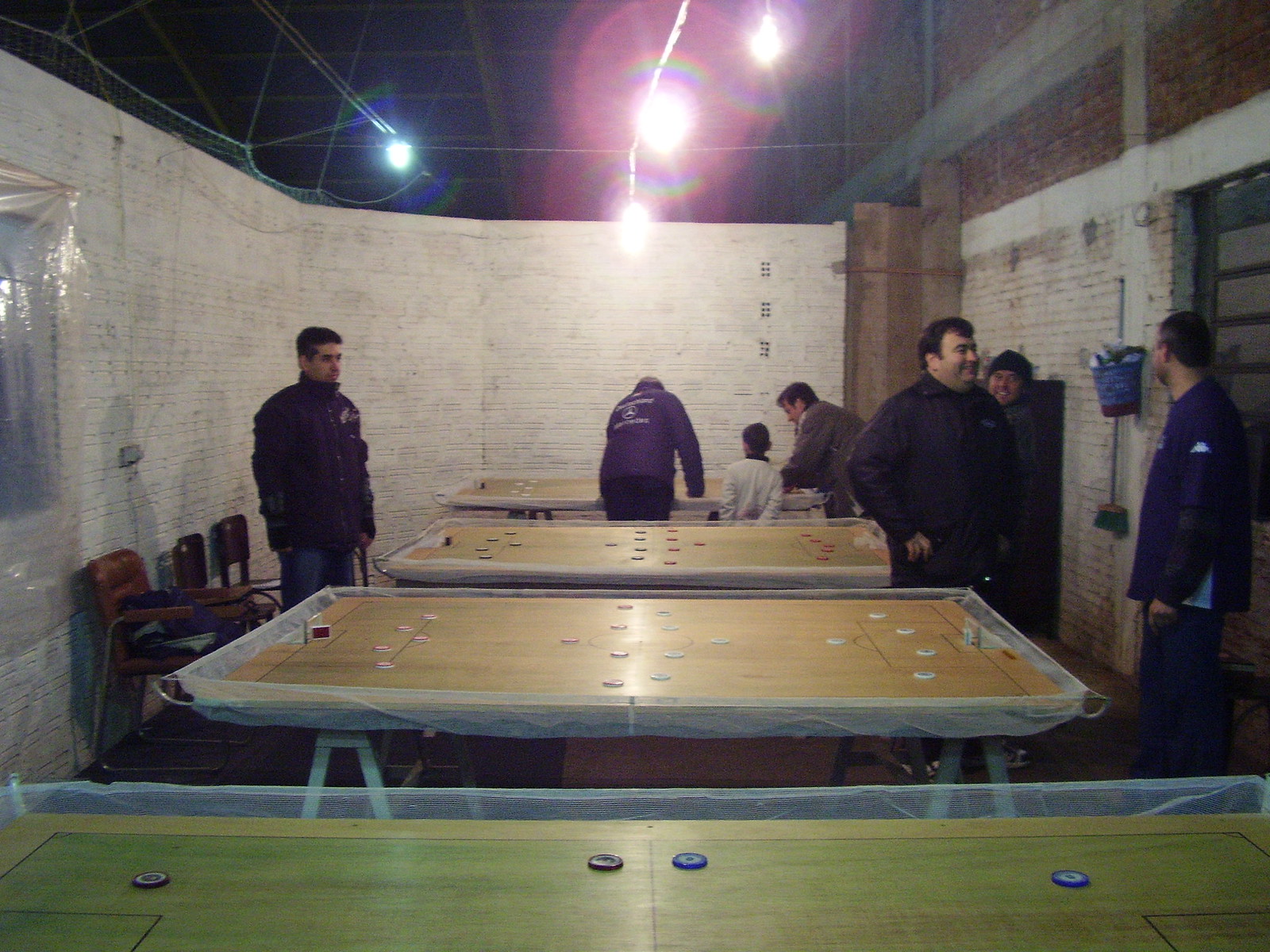In a spacious, white-painted brick room featuring visible rafters and bare light bulbs overhead, seven people, including a child and six adults, are seen around four table hockey games. The tables, which resemble air hockey setups, have white plastic frames and stand on sawhorse-style bases, with brightly colored surfaces and pucks in blue, red, and white. On the right, three men are engaged in conversation, while on the left, a lone man in a dark jacket gazes towards the group, surrounded by three or four maroon chairs. The child and two other adults have their backs to the camera. The room, which appears to be partitioned below a higher ceiling, has a slightly curved, white-painted brick wall and an adjacent dirty white wall with a section of exposed bricks at the top. The scene is vibrant, and although none of the adults are actively playing, some are chatting and laughing.